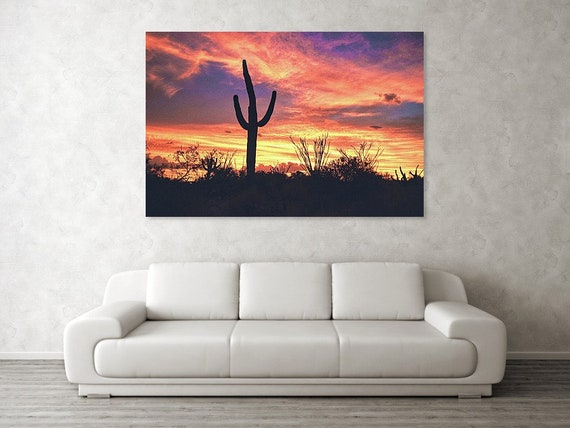The photograph captures an indoor living room scene featuring a white leather couch positioned on a light gray wood-paneled floor. The wall behind the couch is adorned with a cream-patterned wallpaper. Above the three-seat, triple-cushioned couch, a large, vivid painting commands attention. The artwork showcases a striking sunset with a neon orange and yellow sky accented by purple clouds. In the foreground of the painting, there is a silhouette of a tall, cylindrical cactus with two curved limbs and additional silhouetted shrubs, set against the brilliantly lit sky. The overall composition highlights the simplicity and elegance of the white leather couch beneath the vibrant and colorful desert landscape artwork.